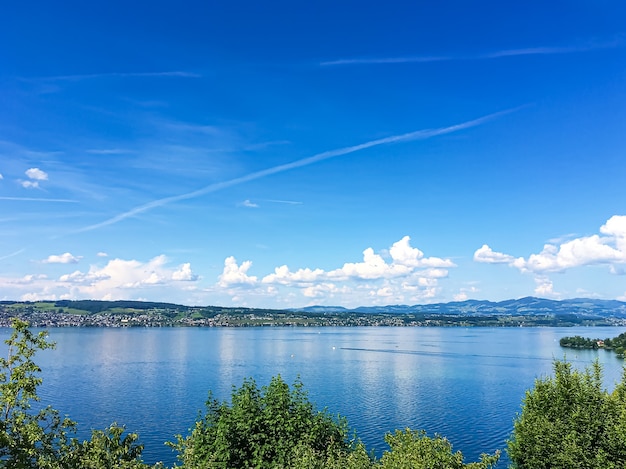A vibrant and serene outdoor scene captures a large, pristine, deep blue lake under a perfect sky. The square, full-color photograph showcases a nearly electric blue sky that lightens toward the horizon, dotted with a few wispy clouds and contrails from passing airplanes. The upper two-thirds of the image is dominated by this beautiful sky, which transitions to thicker clouds near the center. These clouds, along with the azure sky, reflect subtly on the calm lake water, creating a mesmerizing effect accented by tiny ripples. Far off in the distance, the outlines of boats are just barely discernible, while even further, almost imperceptible, are what appear to be buildings or perhaps a cityscape. The bottom portion of the photograph features a thin strip of land with a few scattered trees standing tall. Together, the sky and lake compose a sense of vastness and tranquility, making this scene a captivating portrayal of natural beauty.